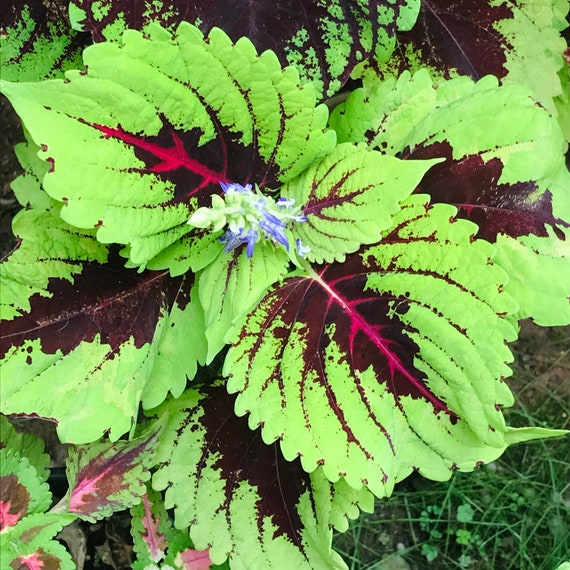This captivating image captures a close-up view of a vibrant begonia plant, showcasing its stunning foliage and delicate flowers. The plant is viewed from above, revealing a central point from which its bright green leaves emanate. Each leaf is detailed with veins of hot pink and edged with a deep, almost black, purple that creates a striking contrast against the lush green. Sprouting from the center, the plant displays small, colorful flowers in shades of bright yellow, violet, and white, with hints of light blue and pink visible at the heart of individual leaves. The image's lower corners show more plant life: in the bottom left, lighter colored leaves with dark pinks, while the bottom right features grassy stems and clusters of small green flowers against a backdrop of regular garden shrubbery and clovers. The overall composition emphasizes the rich, saturated hues of greens, magentas, and purples, portraying a beautifully intricate piece of nature.